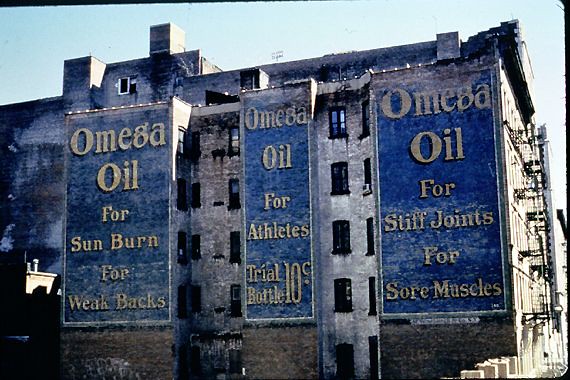This photograph captures the side of an old, weathered building, featuring three large, hand-painted Omega Oil advertisements. The building, made of concrete or brick, is likely situated in a city and appears derelict, with black windows interspersed across its multiple stories. The side of the building, typically hidden by an adjacent structure, is now exposed and utilized for advertising. Each of the three billboards sports a blue background with white text: the left one promotes Omega Oil "for sunburn and weak backs," the middle one "for athletes, trial bottle 10 cents," and the right one "for stiff joints and sore muscles.” The building also has three prominent chimneys on its rooftop. High above, the sky serves as a plain backdrop that emphasizes the antiquated structure’s timeworn appearance.